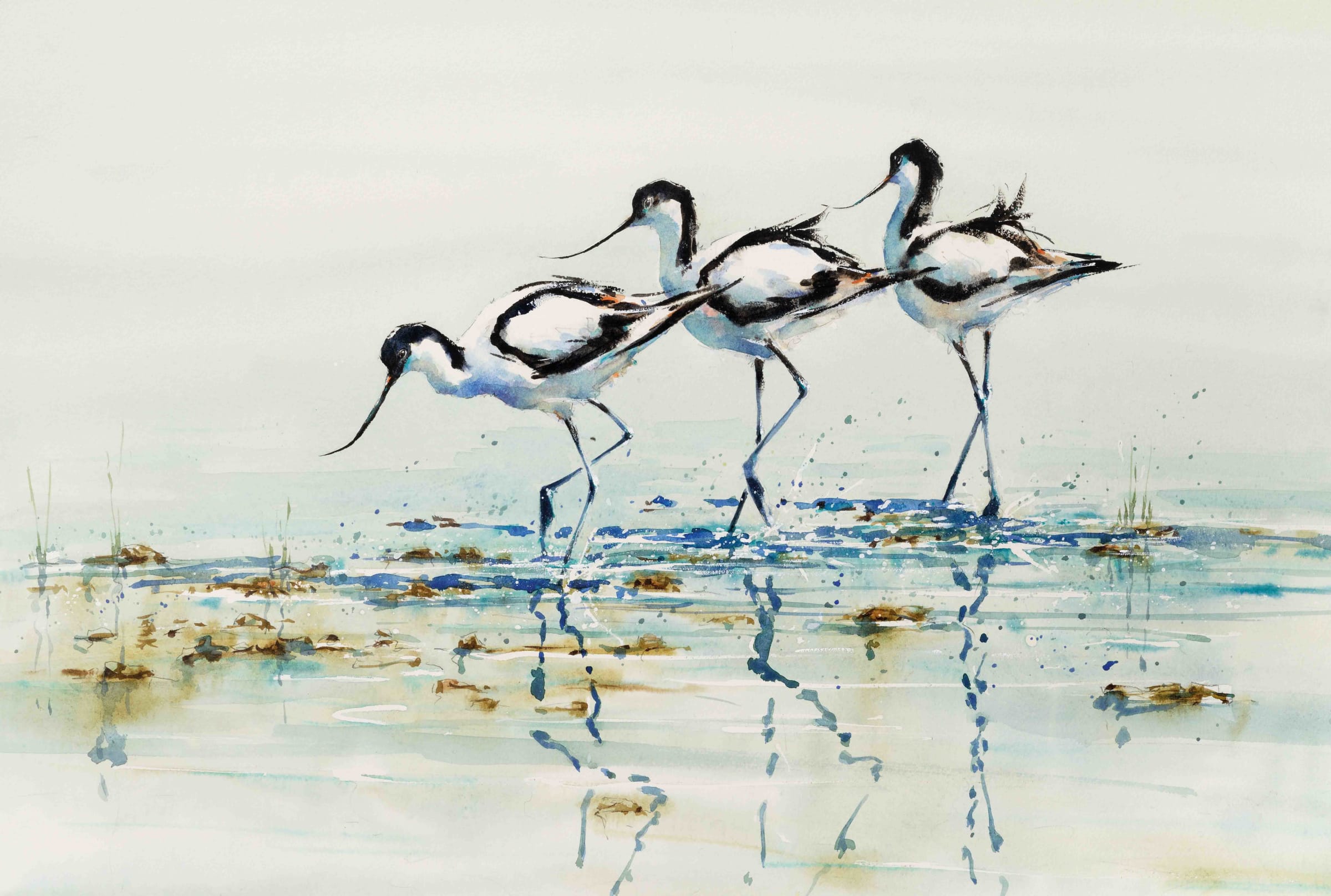This artistic painting illustrates three white birds with black heads, beaks, and detailed black outlining on their wings and tails. They are standing in shallow water, surrounded by some plants and floating logs, with hints of moss scattered on the surface. The first bird on the left, displaying long, slender legs with duck-like feet, is bending down towards the water, seemingly in search of food. Its left leg is raised. The middle bird stands slightly taller and still appears to be bent, gazing into the water with its left leg similarly raised. The third bird on the right stands apart, facing away and looking outward, offering a view more of the back of its head. The birds are centered against an off-white background, and their reflections are visible in the water below them.